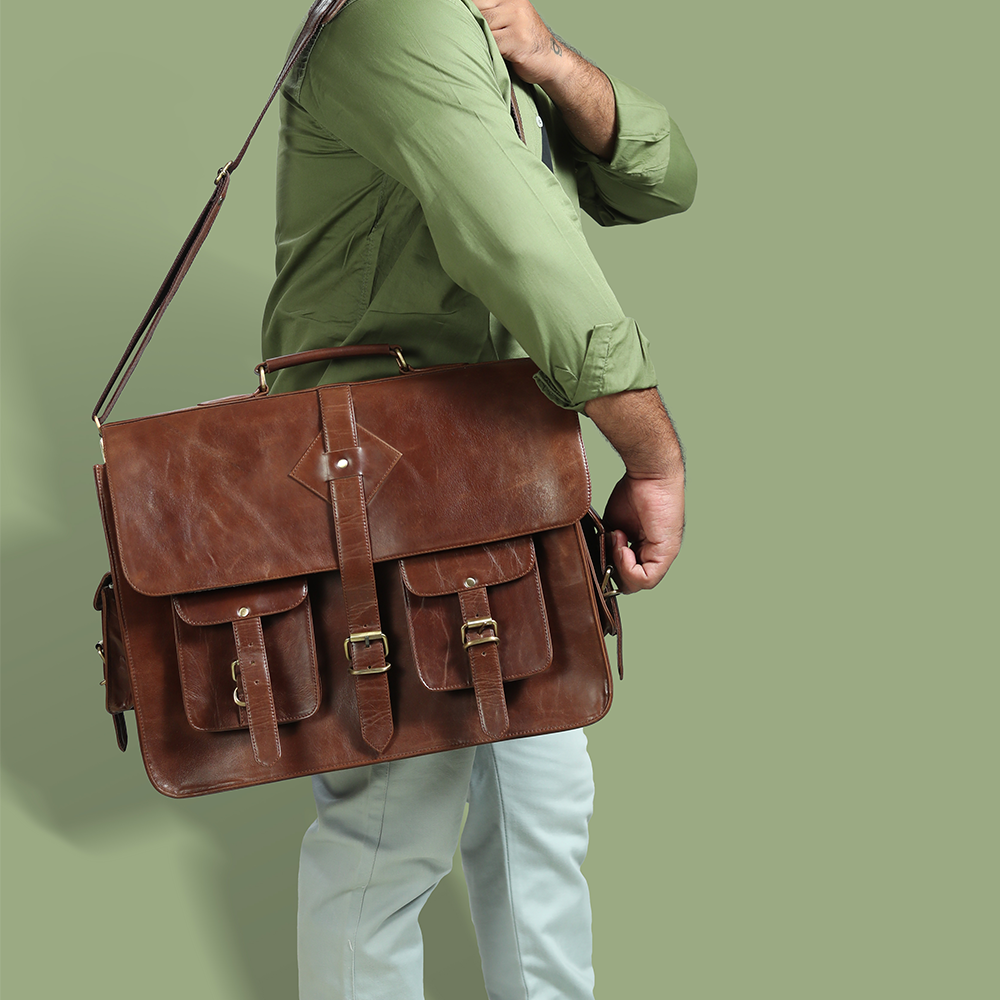This photograph presents a detailed portrayal against a light pale green backdrop, seamlessly matching the hue of the man’s attire. The subject of the image, subtly captured from the side to spotlight his accessory, appears to be a man with hairy arms, adorned in a pale green, long-sleeved, button-up shirt and white pants. His face and shoes are not visible, directing full attention to his sizable brown leather briefcase, which he carries over his shoulder. The briefcase, or satchel, is notably large, exceeding typical briefcase dimensions. It features an intricate design with multiple storage options: one main compartment covered by a flap secured with three vertical gold belt buckles, two front pockets also adorned with buckles, and additional side pockets similarly equipped with belt clasps. The bag blends practical functionality with an ornate decorative touch, with its numerous compartments and imposing presence hinting at its possible use as a laptop case or messenger bag. The overall scene suggests an advertisement, emphasizing the impressive and multifaceted nature of the brown leather briefcase.